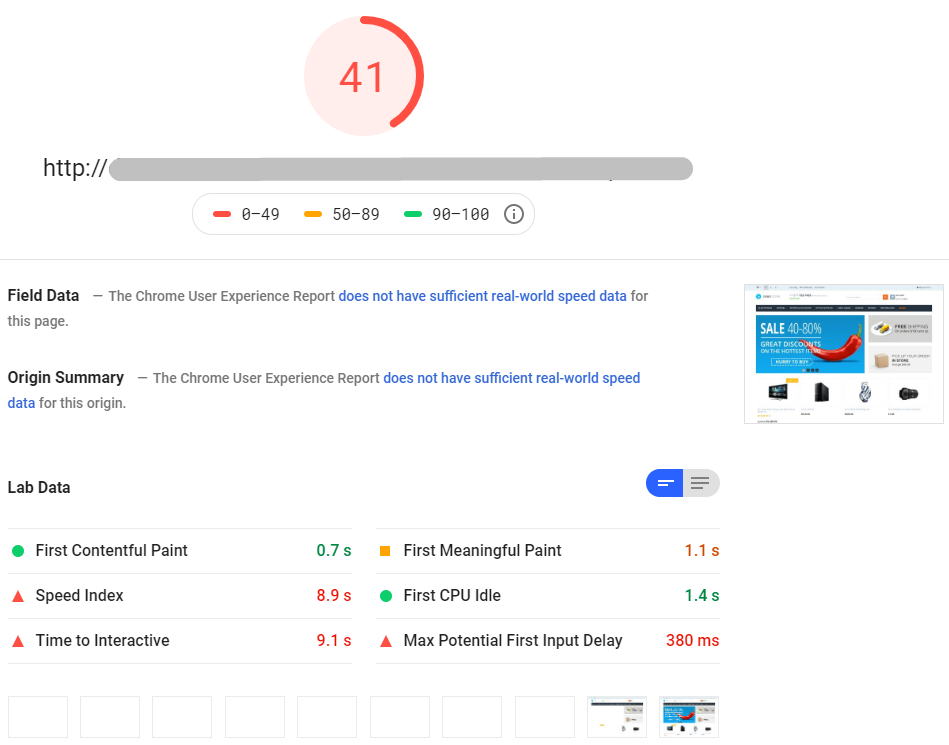This screenshot displays a partial capture of a PC screen, organized as follows:

At the top-center region, there is a very light red opaque circle with a thick red line occupying half of the border on the right side. Within this circle, the number "41" is prominently displayed in red text.

Beneath the circle, a dark grey URL bar is visible, featuring the text "http://" in black on its left side. Below this bar, a thin light grey line outlines a smaller bar with a white background, blending with the screenshot's overall white backdrop. Within this smaller bar, three indicators are present: 

1. A small red line accompanied by the numbers "0-49" in black text.
2. An orange line indicating the range "50-89."
3. A green line, representing "90-100," followed by an information icon shaped like an eye circle.

A thin grey dividing line separates this section from the rest of the page. Below the dividing line, in the top left corner, "Field Data" is written, followed by the explanatory text "The Chrome User Experience Report" in lighter grey. Below this, blue text states, "Does not have sufficient real-world data," with "For this page" in grey.

After a short gap, the text "Origin Summary" appears in black, followed by, in lighter grey, "The Chrome User Experience Report," and again in blue, "Does not have sufficient real-world speed data," concluding with "For this origin" in grey.

Following another short gap, a section titled "Lab Data" is introduced on the left-hand side menu. A very light grey dividing line precedes a two-column list, each containing three items arranged side by side in black text.

**Left-hand column:**
1. "First Contentful Paint" with a green circle to the left and "0.7s" in green to the right.
2. "Speed Index" with a dark orange triangle to the left and "8.9s" in dark orange to the right.
3. "Time to Interactive" with a red triangle to the left and "9.1s" in red to the right.

**Right-hand column:**
1. "First Meaningful Paint" with a dark yellow square to the left and "1.1s" in dark yellow to the right.
2. "First CPU Idle" with a green circle to the left and "1.4s" in green to the right.
3. "Max Potential First Input Delay" with a red triangle to the left and "380ms" in red to the right.

To the right edge of the screenshot, a small banner ad for a PC site is positioned, aligning with the middle of the right border.